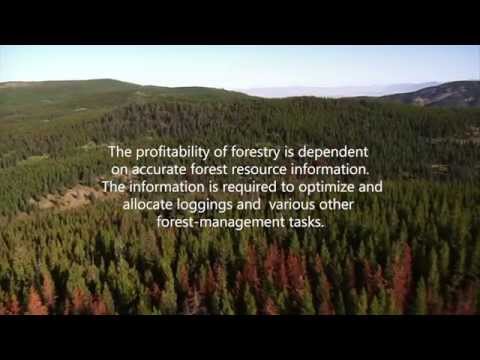This photograph is a rectangular, aerial view of a forest dominated by tall evergreen trees, with some trees showing red-tipped foliage. The image captures a vast, green landscape with rolling, low hills extending into the background, culminating in a pale blue sky with scattered white clouds. Prominent white text at the center of the photograph reads, "The profitability of forestry is dependent on accurate forest resource information. The information is required to optimize and allocate loggings and various other forest management tasks." The text is centered and spans five lines, standing out against the dense forest backdrop. The photograph is framed by thick black bands at the top and bottom, adding a striking contrast to the vibrant natural scenery. A small bare patch of land can be seen on the left, and some mountains in the distance appear bare as well. The overall image suggests a detailed and methodical approach to forest management, underscored by the importance of accurate data.